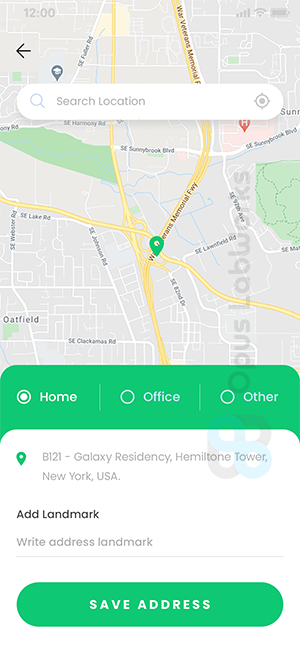The image displays a map interface, with various details illustrating its functionality:

- At the top of the interface, the status indicators show the time (12:00), battery level, Wi-Fi signal strength, and cell signal strength.
- An arrow icon, pointing left, is situated on the top part of the display.
- Below, a prominent search bar is present. It is white with the text "Search location" inside, accompanied by a magnifying glass icon on the left.
- The map itself has a grey background, with prominent yellow streets crisscrossing through the area. White side streets intersect the main roads.
- City names are displayed in larger text, making them easily distinguishable.
- Landmarks are marked with different colored icons. A hospital is designated with a red "H" icon, whereas a green icon marks a specific destination.
- At the bottom of the map, a green banner reads "Home, Office, Other," providing an address: B-121 Galaxy Residency, Hamiltone Tower, New York, USA. The landmark is mentioned alongside.
- The banner includes an option to "Save address" at the bottom, offering convenience for future reference.

The comprehensive design ensures ease of navigation and accessibility for users.